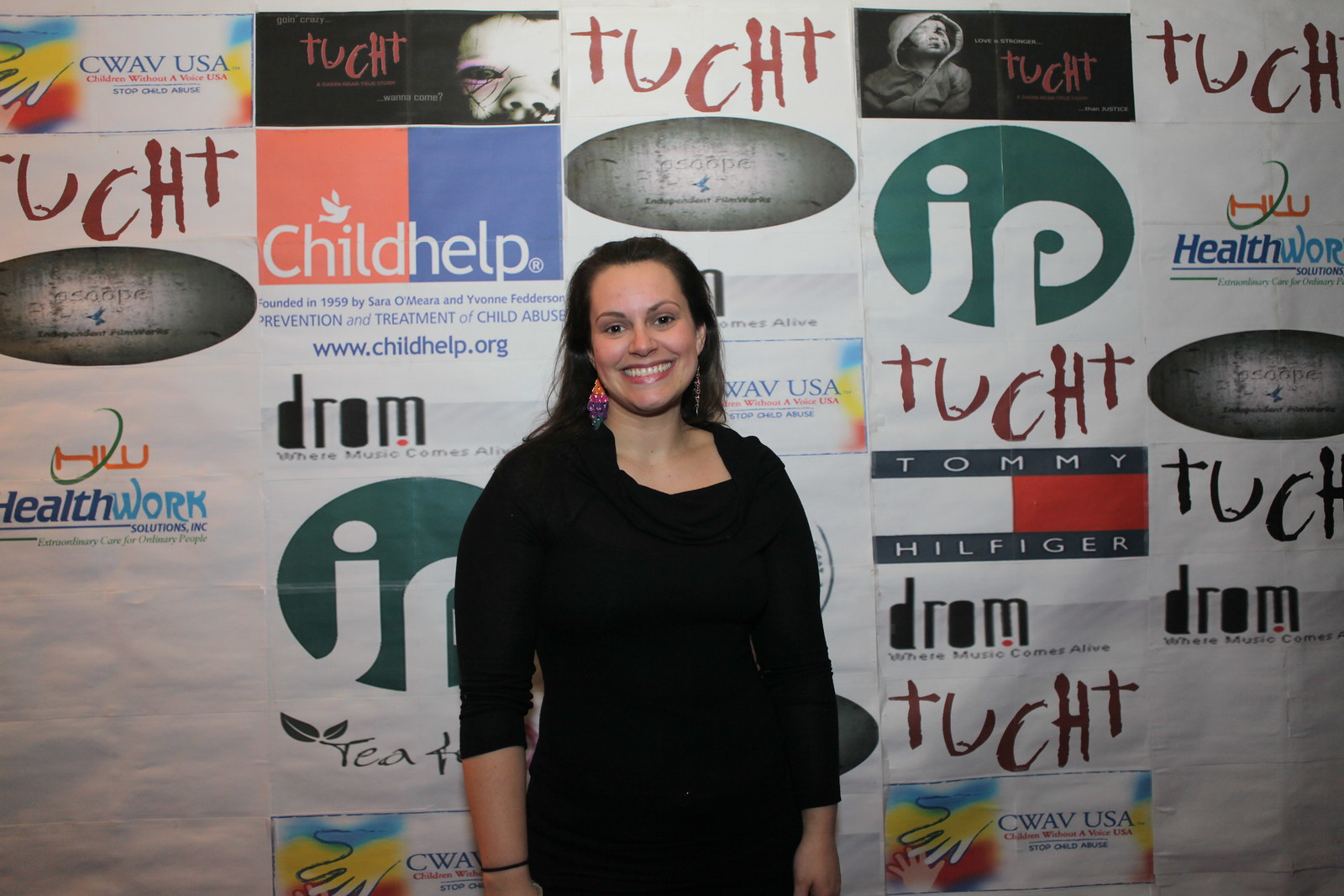This photograph captures a young woman standing at what appears to be an event stage or photograph area, similar to a red carpet setup. She is set against a backdrop featuring various sponsor logos such as Tommy Hilfiger, ChildHelp.org, HealthWorks, IPJP, DROM, TUCHT, and Seaway USA, displayed in a collage on a white banner behind her. The woman is dressed in a black shirt and accessorized with long, diamond-shaped earrings that are colorful, incorporating shades of pink, blue, teal, and orange. Her long black and brown hair is slicked back, and she is smiling broadly for the camera.